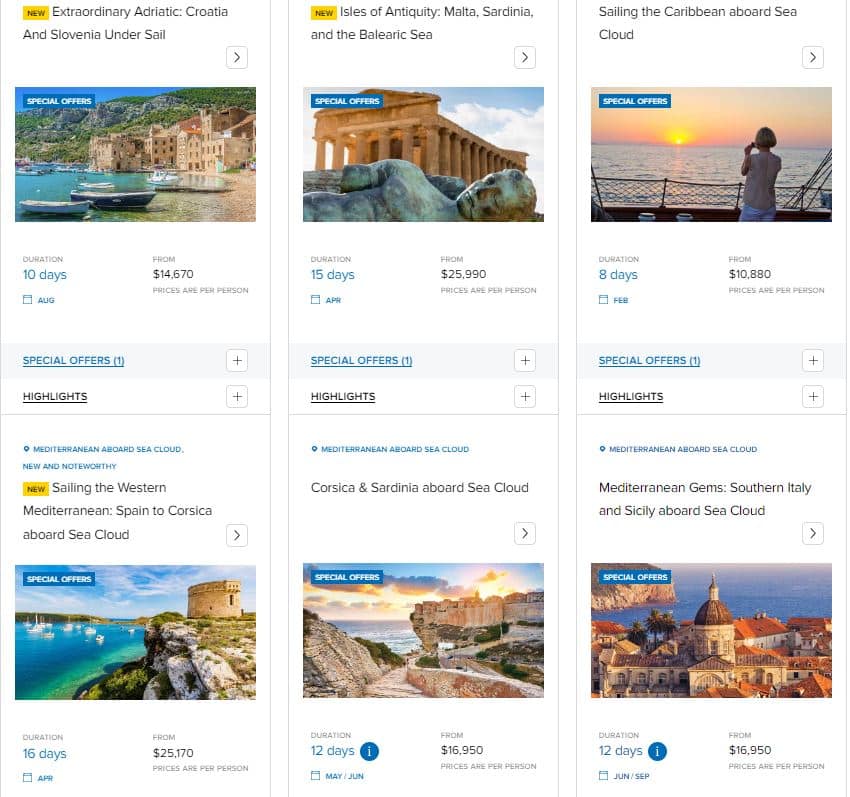This image showcases a collection of six diverse travel offers, organized in a neat grid of vertical white rectangles. Each rectangle contains an enticing travel offer, complete with a descriptive title, an evocative image of the destination, and essential details such as the duration and price of the trip. 

1. **Extraordinary Adriatic: Croatia and Slovenia Under Sail**
   - **Image:** A scenic view of the Croatian coast
   - **Duration:** 10 days
   - **Price:** From $14,670

2. **Isles of Antiquity: Malta, Sardinia, and the Balearic Sea**
   - **Image:** An architectural marvel resembling the Parthenon alongside a toppled ancient statue
   - **Duration:** 15 days
   - **Price:** From $25,990

3. **Sailing the Caribbean Aboard Sea Cloud**
   - **Image:** A serene sunset view captured by a woman standing on the deck of a ship
   - **Duration:** 8 days
   - **Price:** From $10,880

4. **Sailing the Western Mediterranean: Spain to Corsica Aboard Sea Cloud**
   - **Image:** A quaint stone structure perched on a cliffside overlooking a vibrant blue sea
   - **Duration:** 16 days
   - **Price:** From $25,170

5. **Corsica and Sardinia: Above Sea Cloud Aboard Sea Cloud**
   - **Image:** Craggy cliffs rising majestically from the sea
   - **Duration:** 12 days
   - **Price:** From $16,950

6. **Mediterranean Gem: Southern Italy and Sicily Aboard Sea Cloud**
   - **Image:** Not provided in the text
   - **Duration:** Not specified in the text
   - **Price:** Information not fully detailed in the text

Each offer tantalizes with unique experiences, promising memorable journeys to some of the world's most picturesque and culturally rich locations.